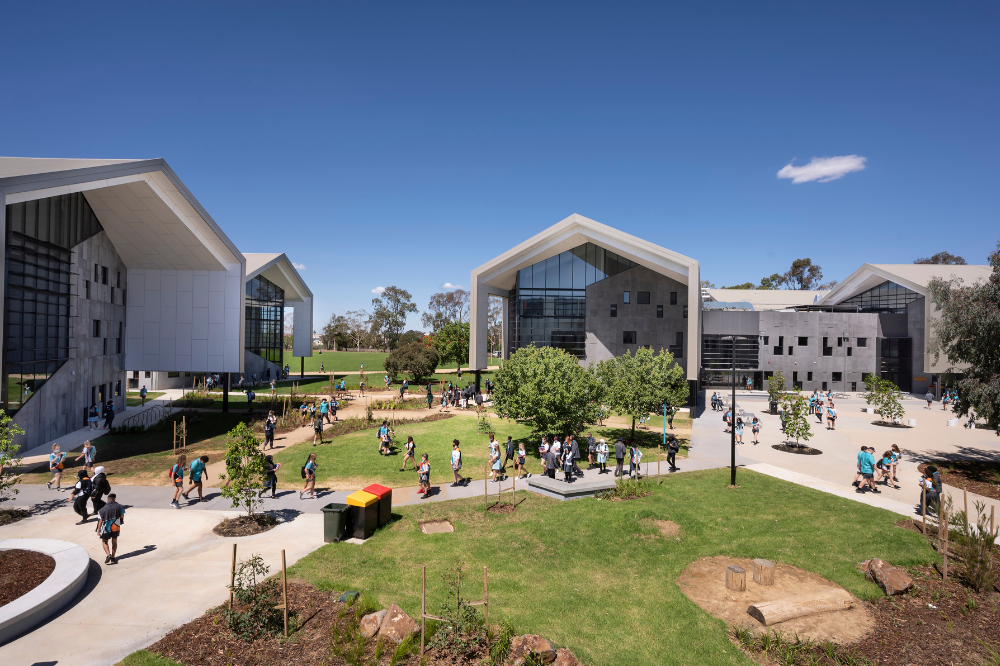This aerial photo captures a vibrant campus, possibly for a college, summer camp, or high school, bustling with activity under a beautiful blue sky adorned with a single white cloud. The image prominently features three modern buildings with slightly hexagonal, pointed white roofs and dark gray, paneled walls interspersed with many windows, including glossy panes below the roofs. These buildings are arranged at the top of the image, with numerous pathways connecting them and filled with children or young adults predominantly dressed in blue t-shirts, shorts, and running shoes.

In the foreground, several garden beds with stakes for growing plants are visible, leading into a circular tan ground area. This area features logs arranged to resemble a mediocre smiley face. Adjacent to these garden beds is a large concrete lot with three trash cans—one without a lid, another with a yellow lid, and a third with a red lid. The space is well-landscaped, boasting lush green grass patches, healthy trees, and ample open areas where people are walking, congregating, and enjoying the outdoors.

The scene captures a moment of lively interaction and movement, set against the backdrop of flourishing greenery and a patch of meadow, indicating a harmonious blend of nature and modern architecture.